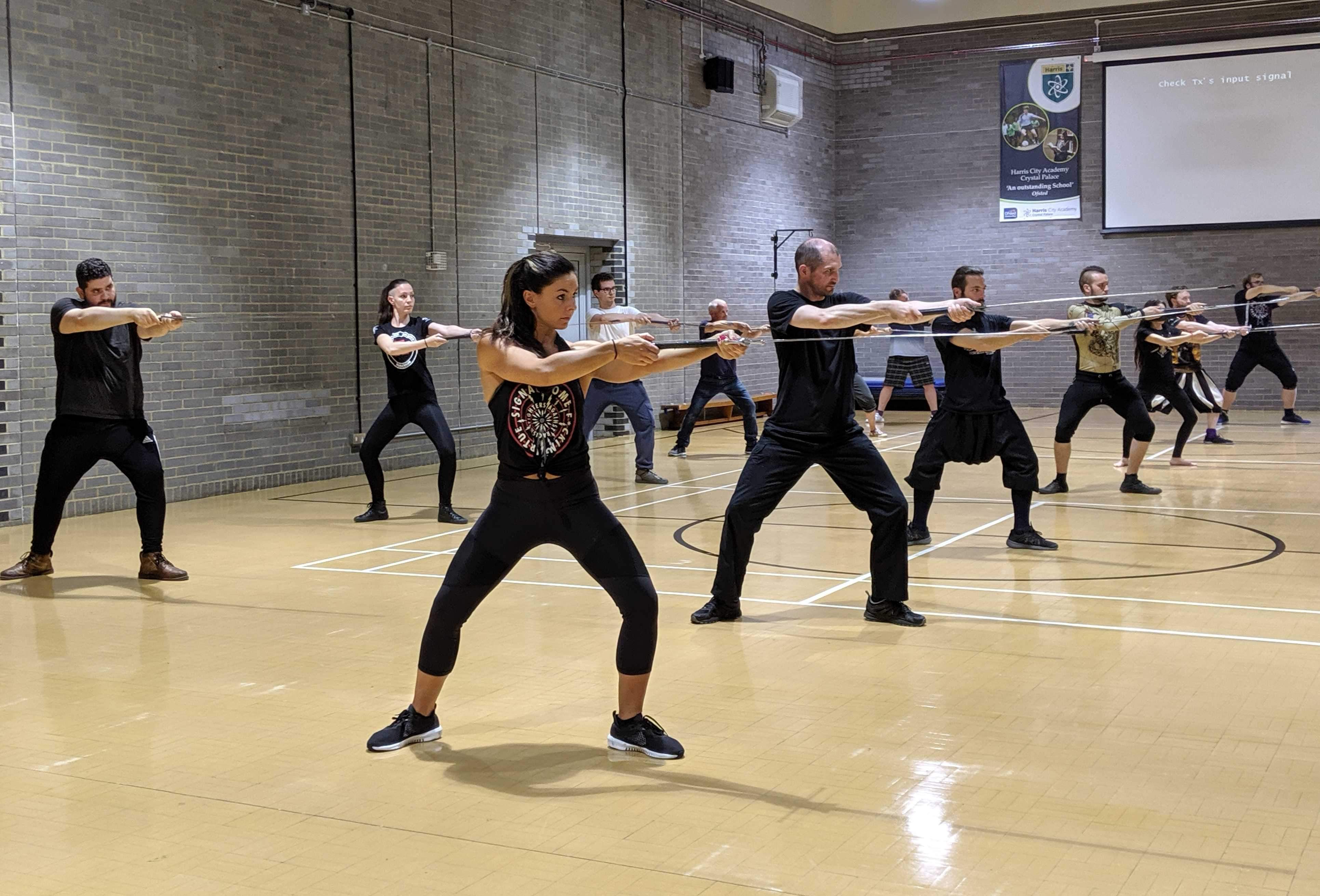In this detailed image, a group of men and women are engaged in what appears to be a choreographed exercise or self-defense class in a spacious indoor setting. They are positioned on a tan-colored court, which might be a gymnasium, marked with distinctive white and black tape lines and circular patterns. The participants are organized into two lines angled towards the right, each holding thin poles with black handles in front of them, possibly for a synchronized activity or preparation for a performance. 

Notable among the group is a woman slightly off-center to the left, wearing a black top with a large insignia, black sweatpants, gray tennis shoes, and sporting black hair. The background reveals a gray brick wall, extending from the left side into the middle and upper right portion of the image. Dominating the upper right corner, there is a white projector screen accompanied by a blue banner adorned with information and logos. Additional details include a prominent black speaker and a white device mounted on the wall, contributing to the room's multi-functional ambiance.